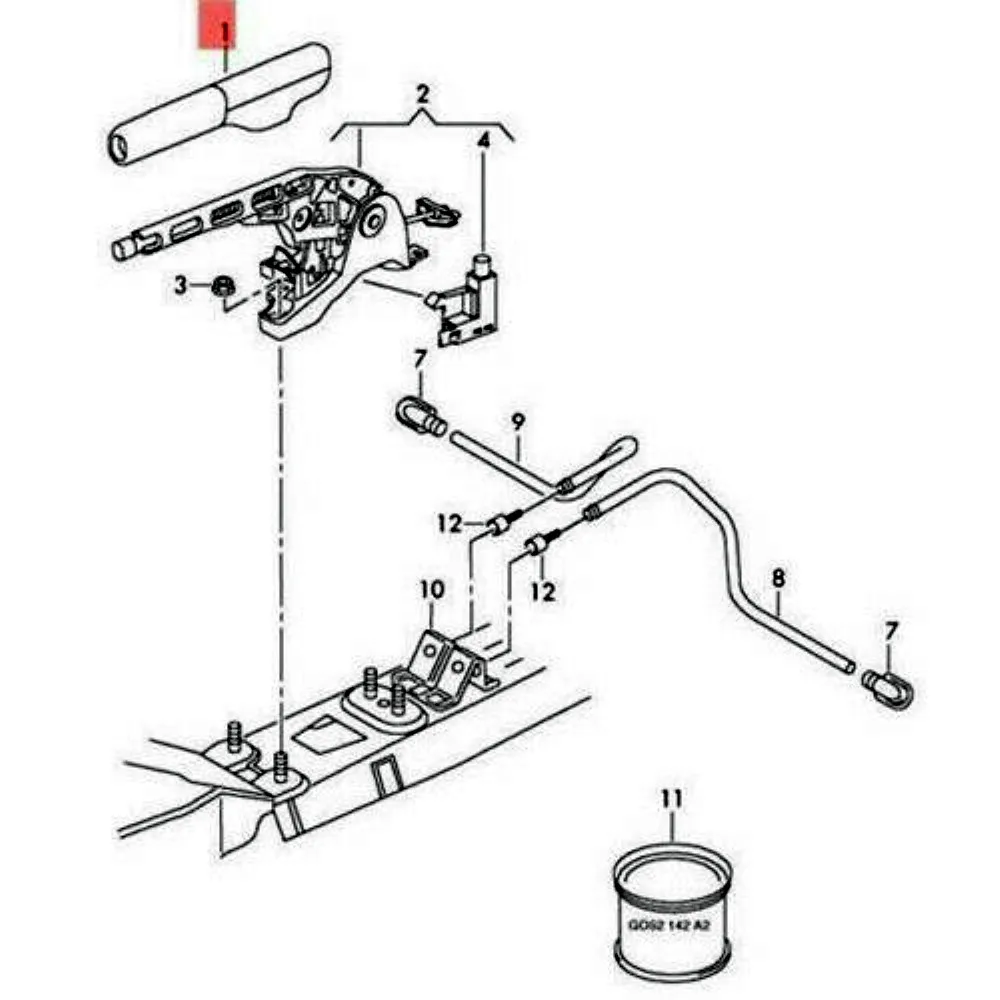The image is an infographic appearing to be a black and white schematic from an instruction manual, likely related to a mechanical device such as a car, boat, or potentially a gun. The drawing details various components, labeled with numbers 1 through 12, with each part depicted in basic black lines against a white background. Component number 1 stands out with a red rectangle around its label, distinguishing it from the others. This part appears to be a tube situated at the top of the diagram. Other notable features include a complicated assembly labeled with numbers 3 and 4, which seems attachable to a panel below, and two curved tubes connected to a metal bar, each secured with screws. Additionally, component number 11, resembling a tin can or round cylinder, is positioned at the bottom of the schematic. The diagram is devoid of any color beyond the black and white lines and the single red rectangle, emphasizing its function as a straightforward technical illustration.